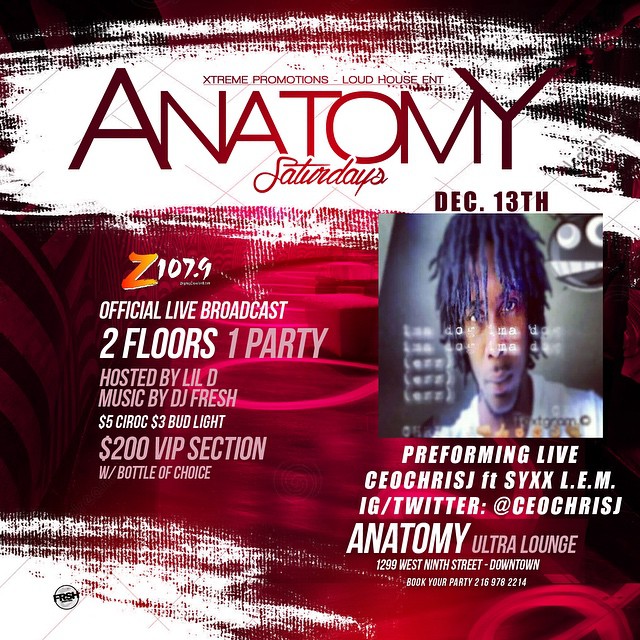This promotional flyer for "Anatomy Saturdays" presents an event taking place on December 13th, advertised by Extreme Promotions and Loud House ENT. The event features an official live broadcast by Z107.9 and promises "Two Floors, One Party" hosted by Lil D with music by DJ Fresh. Highlights include $5 Ciroc, $3 Bud Light, and a $200 VIP section with a bottle of choice. The red and black-themed background sets the stage for a night of vibrant entertainment. On the right side, an African-American man with medium-length dreadlocks, colored purple or blue in the front and darker at the back, is depicted in a headshot. He's wearing a white t-shirt and is introduced as performing live, listed under the name CEO Chris J, with social media handles @SilkReichG on IG and Twitter. The venue is the Anatomy Ultra Lounge located at 1299 West 9th Street, downtown. The flyer encourages booking your party at 216-978-2214 and features a watermark with the letters FRSH inside a black circle on the bottom left.